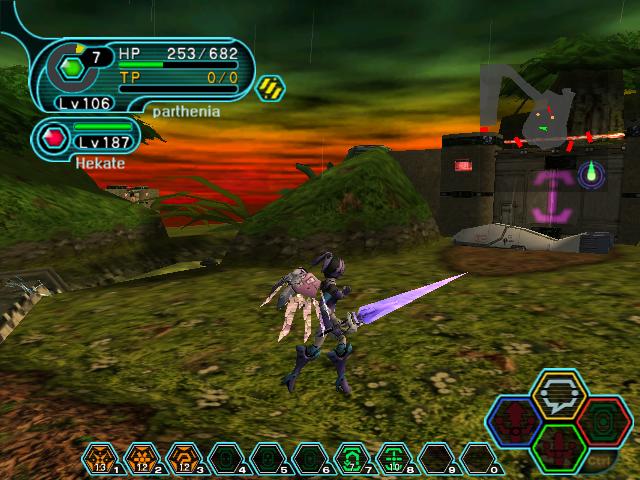A detailed in-game screenshot from a futuristic fighting video game. The large, square image prominently features the main character, wielding a massive sword, accompanied by a small, white crab-like creature serving as her sidekick. They are traversing a lush, grassy landscape adjacent to a daunting fortress, complete with firmly shut metal doors. At the top of the screen, a blue oval interface displays critical information such as hit points, total points, and both the character's and sidekick's levels. The bottom of the screen houses an action bar for quick access to abilities and tools, while the bottom-right corner includes an options bar for chatting with other players and managing inventory. The overall scene exudes a futuristic vibe, blending elements of adventure and strategy.